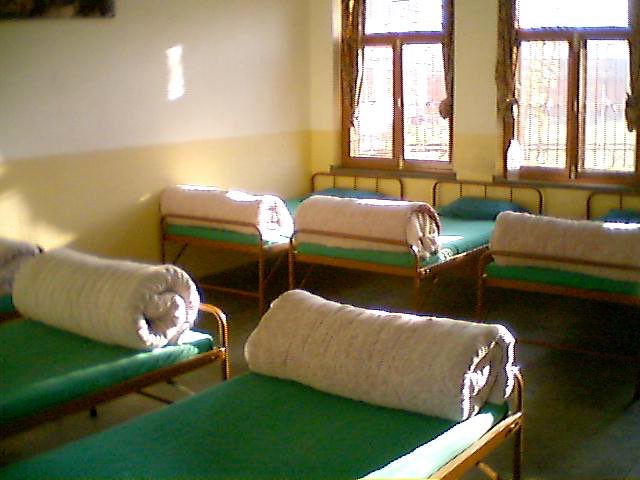The image depicts a brightly lit, basic dormitory room, likely from a boarding school or children's home, characterized by its minimalistic setup. The room contains six identical twin-size beds with medium brown wooden frames, each outfitted with a very thin green mattress, a pillow or rolled-up blanket at the head, and a tan blanket neatly rolled up at the foot. Sunlight streams in through two windows on the right side of the room, which feature brown wooden frames and sheer brown curtains. The walls are painted with a simple color scheme – the bottom half yellow and the top half white, divided by a horizontal line. The photograph captures the room from a corner perspective, looking diagonally towards another corner, revealing the orderly arrangement of the beds and the gray cement floor. The overall atmosphere suggests a functional and austere environment, evocative of the 1960s or a utilitarian institution.